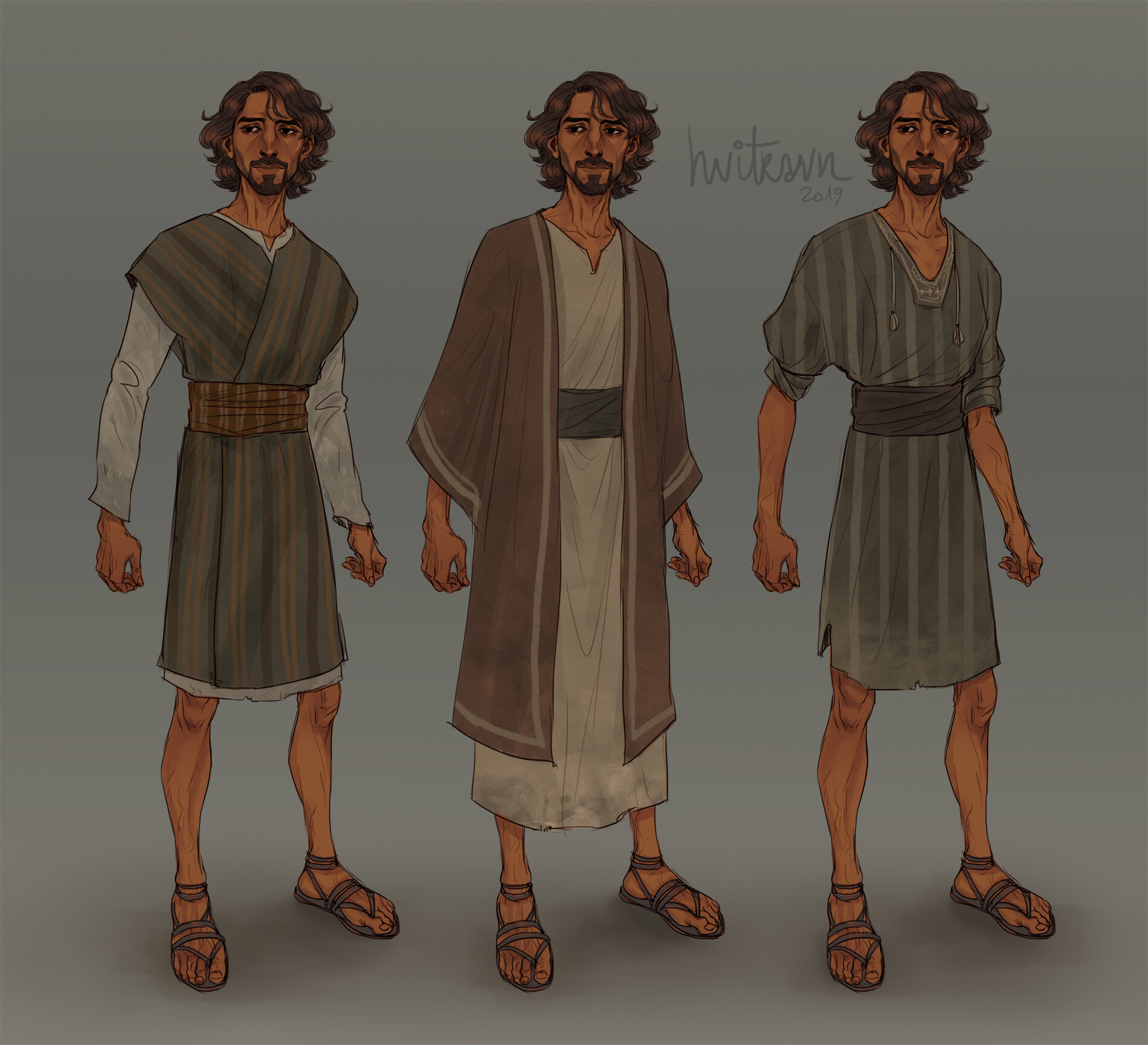The image depicts concept art for a character that resembles an ancient peasant, potentially from biblical times. The character appears three times in identical poses, each with variations in clothing. The man is thin, has short, curly brown hair, a goatee, and is wearing tied sandals. The setting is against a gray background, and the drawings have a hand-drawn, cartoonish style.

In the leftmost image, the man wears a long-sleeved white undershirt beneath a robe that features green and brown stripes, cinched at the waist with a belt. The middle depiction shows him in a skirt-like garment with a black belt, a brown overgarment with long sleeves, and stripes down the sides. The final image on the right shows him in a knee-length green shirt with light green stripes down the center, an open V-neck collar, and rolled-up sleeves, also fastened with a belt around the hips. Each outfit reflects a different style, reminiscent of attire from the times of Jesus Christ, with distinct robe variations and sash details. All three renderings emphasize his sandals and the gray background.